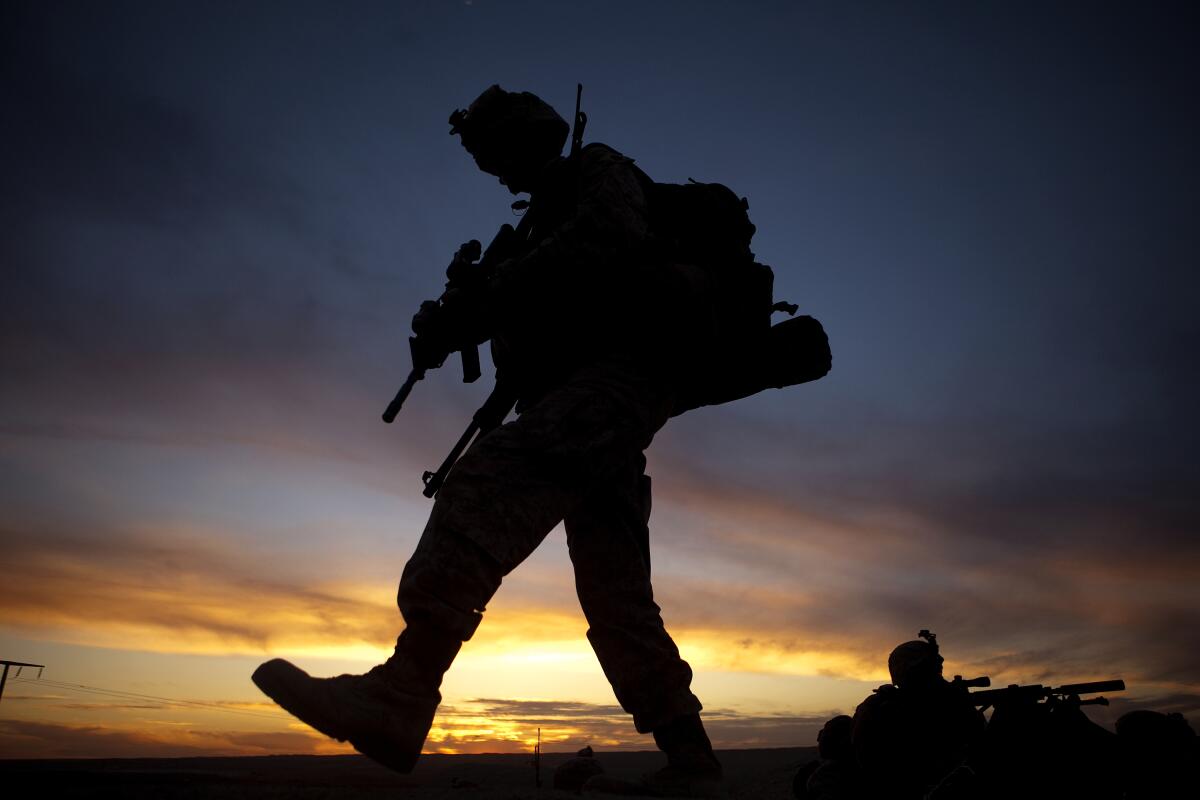The photograph captures a striking silhouette of a soldier, prominently centered and viewed from a low angle, giving an impression of grandeur against the dark twilight sky. The soldier, identifiable only by his outline, is encumbered with a large, heavy backpack and standard military gear, including armor and a helmet. He holds a machine gun pointed down as he marches through a dry field. The setting sun casts deep shadows, rendering all features in stark black, with just a hint of purple and blue in the sky, and a golden light peeking through the distant horizon. To the bottom right, other soldiers are visible, similarly silhouetted, some with long rifles, potentially snipers, in hand, appearing alert and poised, directing their gaze and weapons into the distance. A solitary pole stands near the lead soldier’s boot area, adding to the barren and desolate feel of the scene. The overall mood is one of solemnity, focus, and hidden potential under the cloak of twilight.